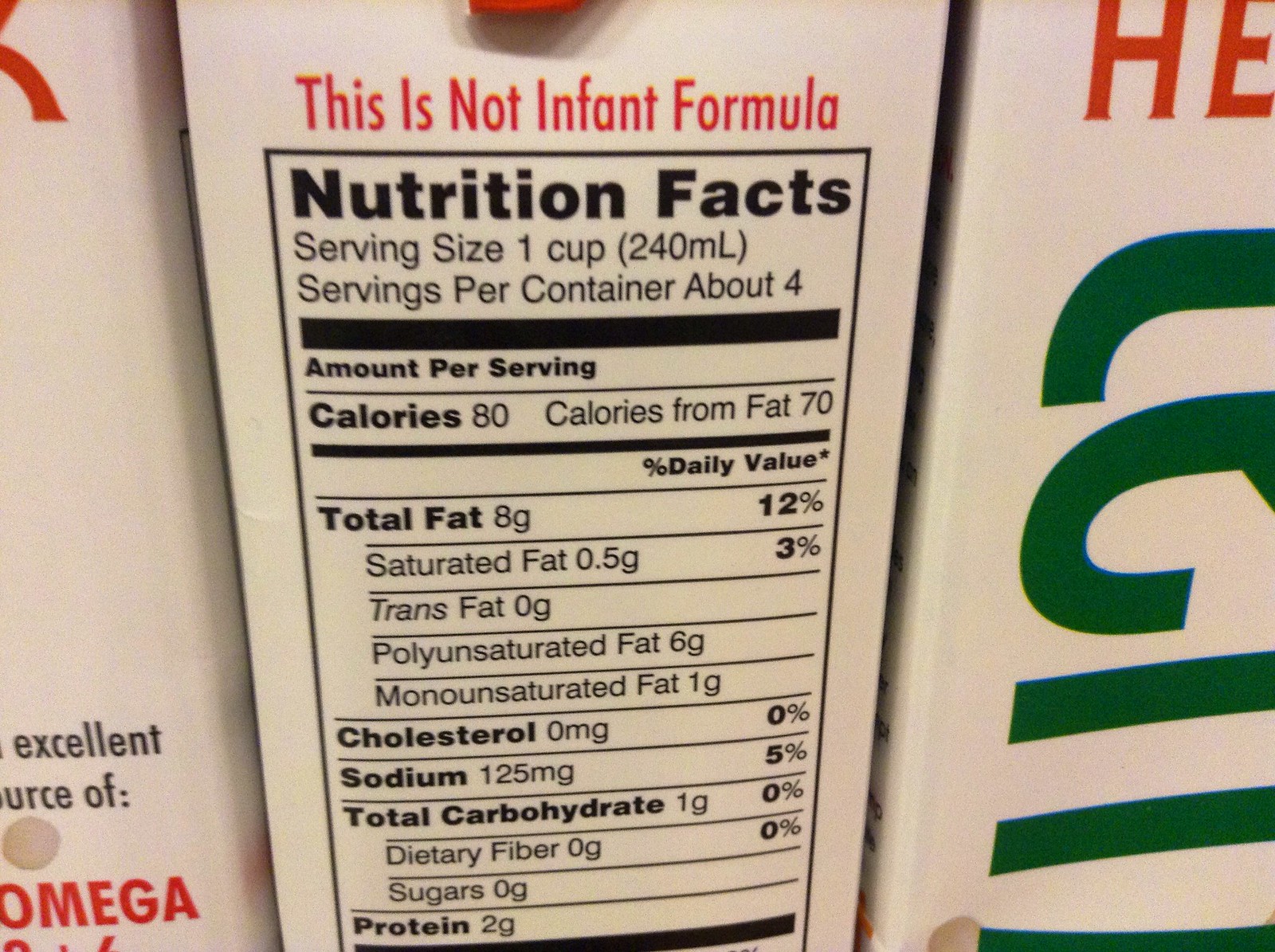This image features a close-up of a Nutrition Facts label on the side or back of a rectangular, white carton. Dominating the top in bold red text are the words "This is not an infant formula," immediately drawing attention. Below that, in the main section, the label specifies the serving size as 1 cup (240 milliliters), with about 4 servings per container. Each serving contains 80 calories, with 70 calories from fat. The detailed nutritional breakdown highlights 8 grams of total fat (including 0.5 grams of saturated fat, 0 grams of trans fat, 6 grams of polyunsaturated fat, 1 gram of monounsaturated fat), 0 milligrams of cholesterol, 125 milligrams of sodium, 1 gram of total carbohydrates (0 grams of dietary fiber and sugars), and 2 grams of protein. To the left of this central Nutrition Facts label, there's a partially visible section of another similar-looking container, with the word "Omega" prominently in red lettering at the bottom, hinting at its nutritional benefits. The white background and the straight edges of the carton imply a standard rectangular shape, likely for a milk or cream product.